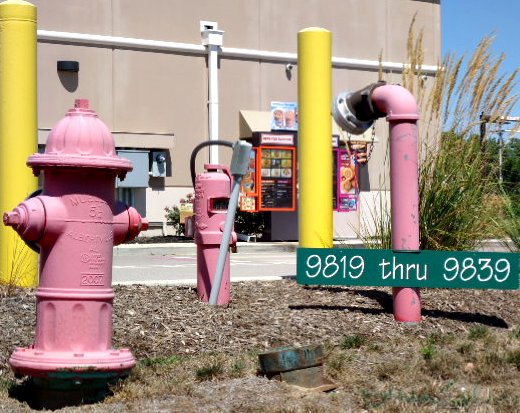The image depicts a detailed outdoor scene near what appears to be a fast-food drive-through adjacent to a tan, warehouse-style building. In the foreground, there is a reddish-pink fire hydrant situated on an area covered with wood chips and surrounded by grass. To the right of the hydrant, there is a pink curved top fire department standpipe with a green sign, bearing white text that reads "9819 THRU 9839." Further right, there is another standpipe, presumably for utilities access, and a gray conduit with a silver metal box. Two yellow metal poles act as barriers in front of the standpipes, likely to prevent damage from vehicles. 

In the background, the tannish building features white gutters across its center and a brown, triangle-shaped security light box. There are also two security cameras and an electrical box visible. The building appears to have a drive-through with a brown and red-outlined menu board, displaying images of food and summer frozen drinks. The drive-through area is framed by weeds, plants, and saltwater reeds, which are tall and feather-like. Above the scene, the sky is blue, with parking lot lights and trees positioned further back, adding to the environmental detail.